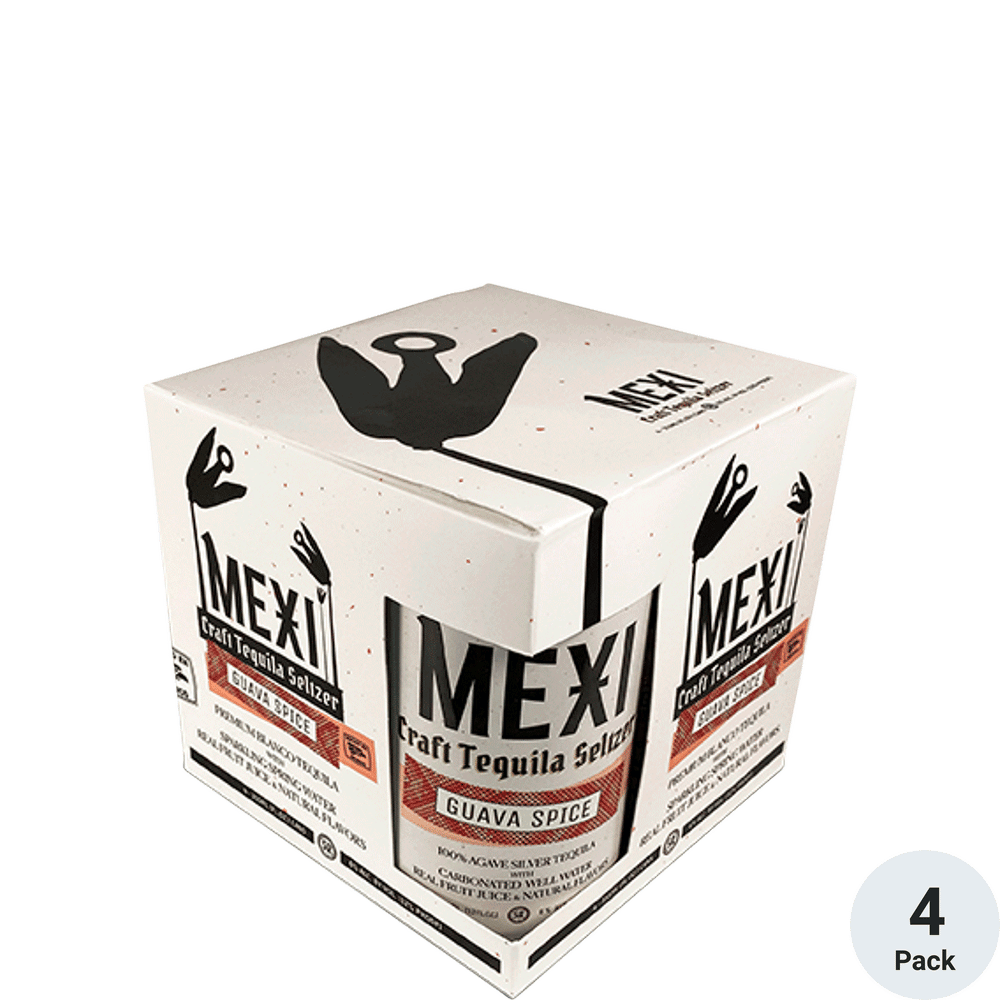In this close-up image, we focus on a compact, mostly white box containing a four-pack of Mexi Craft Tequila Spritzer, showcasing the flavor 'Guava Spice.' Dominating the design is the brand name "M-E-X-I" in bold black lettering, with a distinctive cross bar across the center of the 'X'. This lettering is prominently featured against a black bar that also holds the product description "Craft Tequila Spritzer." Below this, additional black text indicates the flavor 'Guava Spice'. The box features a cut-out corner revealing one of the cans inside, sporting the same branding elements. Both the box and the can highlight the ingredients "100% Agave" and "Carbonated Well Water." The box is further detailed with sleek black illustrations, resembling either a bird silhouette or flower petals. There's also a circular emblem on the right side of the box with the text "4-Pak" inside. Additional information about the product and the company is scattered across various parts of the packaging.